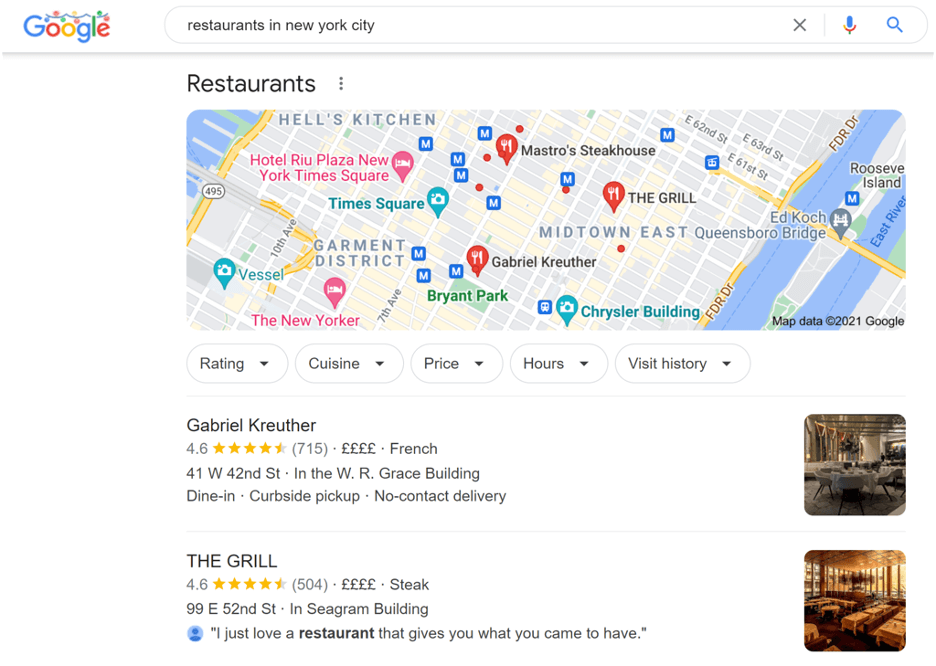A search for "restaurants in New York" was conducted, evident from the Google homepage adorned with festive Christmas lights. The search results are displayed against a white background and focus on the areas surrounding Hell's Kitchen and the Garment District. A map pinpoints various dining options, including Gabriel Kreuther, which boasts a 4.6-star rating and is considered very expensive, indicated by four pound signs (££££). This French restaurant, located in the W.R. Grace Building, offers dine-in, curbside pickup, and no-contact delivery options. The imagery reveals a plush, comfortable interior with inviting tables and chairs.

Another highlighted establishment is The Grill, which also garners a 4.5-star rating and four pound signs (££££), emphasizing its high price point. Known for its steak, The Grill is situated in the Seagram Building and is renowned for providing exactly what patrons crave. A review underscores the satisfaction of enjoying their signature dish. The restaurant features a panoramic view of New York, likely from an upper floor, as indicated by its window-lined setting.